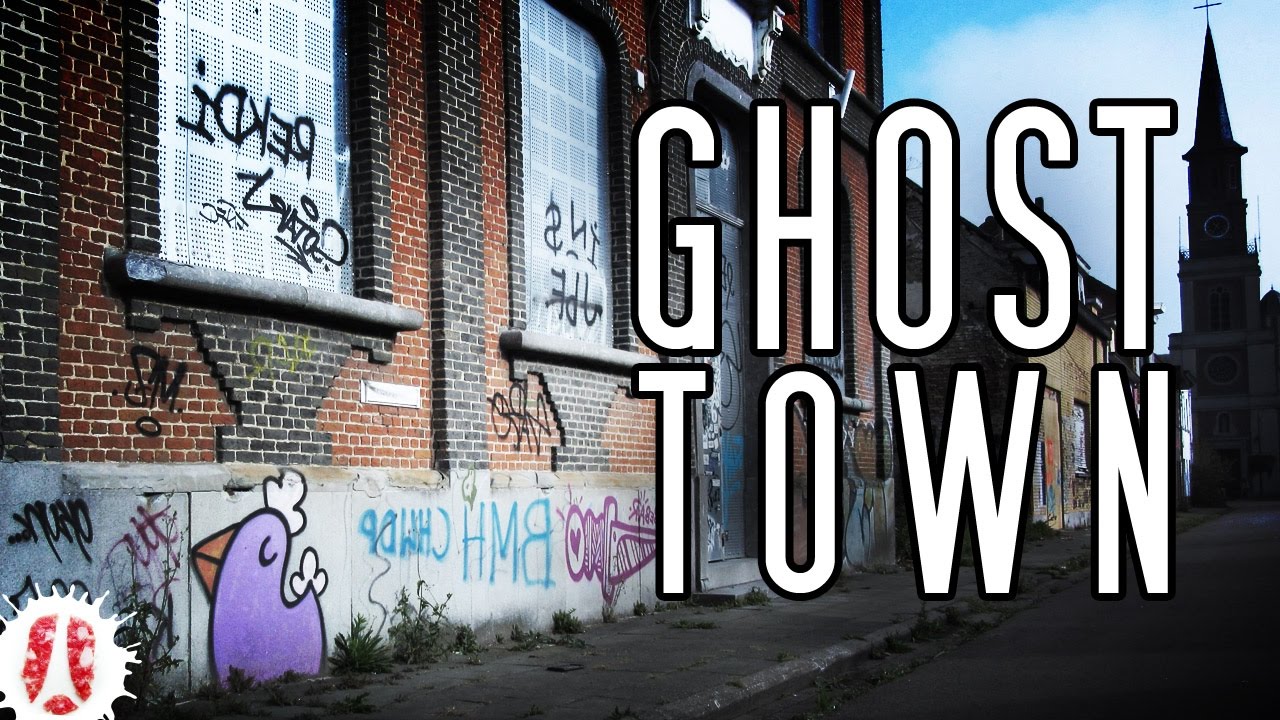In this color photograph of a ghost town, the viewer's attention is immediately drawn to the large white text outlined in black, occupying nearly the entire right half of the image. This bold, narrow font prominently announces "ghost town" over a backdrop of an eerily deserted street. 

On the left side of the photo stands an old, abandoned brick building, composed of black and red bricks. The building is covered in vibrant graffiti, showcasing a mix of black, purple, and blue hues. Among the various tags and names, a purple cartoon character resembling a whale with a small hat, as well as what appears to be a purple bird or chicken, catches the eye. The windows of the building have a peculiar white grid pattern, suggesting they may have been boarded up. Both the sidewalk running along this row of abandoned buildings and the street itself are visible, with the sidewalk noticeably overgrown with green weeds sprouting through its cracks and edges.

In the distance on the right side, partially visible behind the imposing text, is an old and possibly abandoned church or city hall. This stately building features a clock tower and a spire, although it is cloaked in shadow and appears darkened. The street itself is a silent expanse of black asphalt, devoid of any cars, contributing to the desolate atmosphere. Detailing the bottom left corner is an indeterminate white splat or logo, adding another layer of mystery to this haunting urban scene.